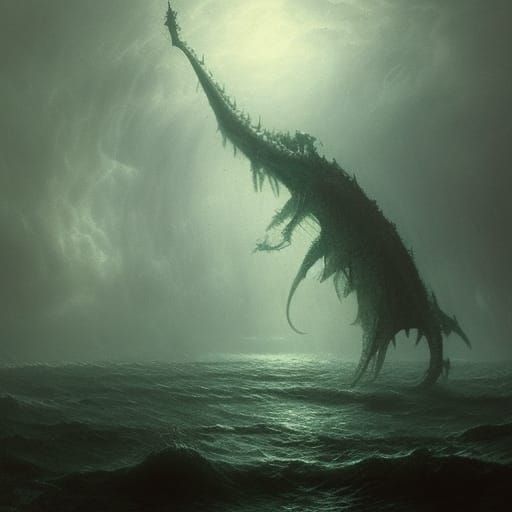This vertical rectangular image depicts a fantastical, otherworldly scene at sea, bathed in an eerie greenish tint. The perspective places you amidst dark, tumultuous waves, which hint at the depth and vastness of the ocean beneath. The scene is set under a stormy, cloud-filled sky, casting a turbulent halo with a hazy spot of light near the top center, possibly the sun or moon peeking through. Rising ominously from the bottom right and extending to nearly the top of the image is a giant, tentacled creature, reminiscent of a monstrous, worm-like entity. Its thick, plant-covered body writhes with multiple tentacles, and it terminates in a long, thin neck with a tiny, cylindrical head. The overall atmosphere is dark, with the creature’s silhouette stark against the chaotic backdrop, conjuring a sense of unease and otherworldly presence.